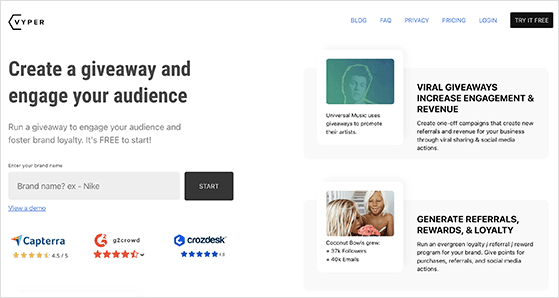The image is a left-to-right horizontal screenshot capturing a webpage, which can be accessed via a computer or smart device. The background of the site is primarily white, framed by a thin black line along the edges. In the upper left-hand corner, the site's branding is evident with the word "Viper" alongside a small emblem.

On the upper right-hand corner, there is a blue navigation menu featuring options like "Blog," "Frequently Asked Questions," "Privacy," "Pricing," "Login," and a prominent black button labeled "Try it Free," though this area appears slightly blurry.

The page's main content starts on the left side with bold black text that reads, "Create a giveaway and engage your audience," followed by an explanatory sentence, "Run a giveaway to engage your audience and foster brand loyalty. It’s free to start." Below this, there is a box prompting users to "Enter your brand name" with an example like "Nike," and a "Start" button for initiating the process. Additionally, users can choose to view a demo.

Further below, there are star ratings and reviews from "Capterra," something in red, and "Craw's Desk." On the right side of the page, there are clickable articles with accompanying images, offering more detailed information.